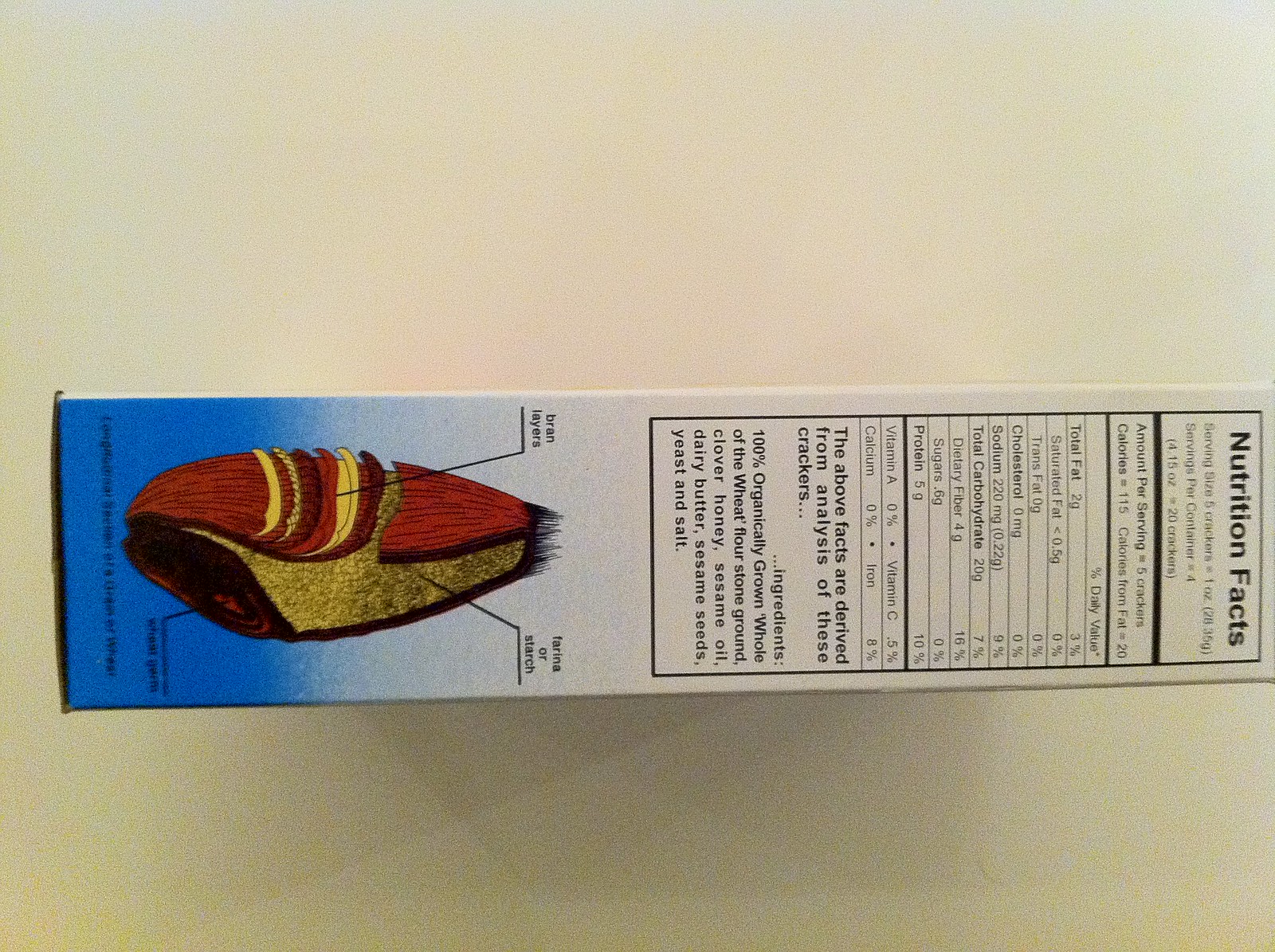The image features a light beige background with a cereal box positioned horizontally, displaying its nutrition panel prominently facing the camera. The bottom part of the box is on the left, while the top part extends to the right. The left side of the box is distinguished by a vibrant, deep blue section that transitions into the white spine area of the rest of the box. On this blue background, as it melds into the white, there is an illustration of a wheat kernel laying on its side. The kernel is split open, revealing the bran and wheat germ areas, which are detailed with various dark lines and labels pointing to specific parts of the grain. The upper right section of the box features the start of the nutrition panel. This area, located on the top right side of the box, has "Nutrition Facts" written in bold black letters, followed by the familiar format of black nutritional information text on a white background, providing detailed nutritional data of the cereal product.